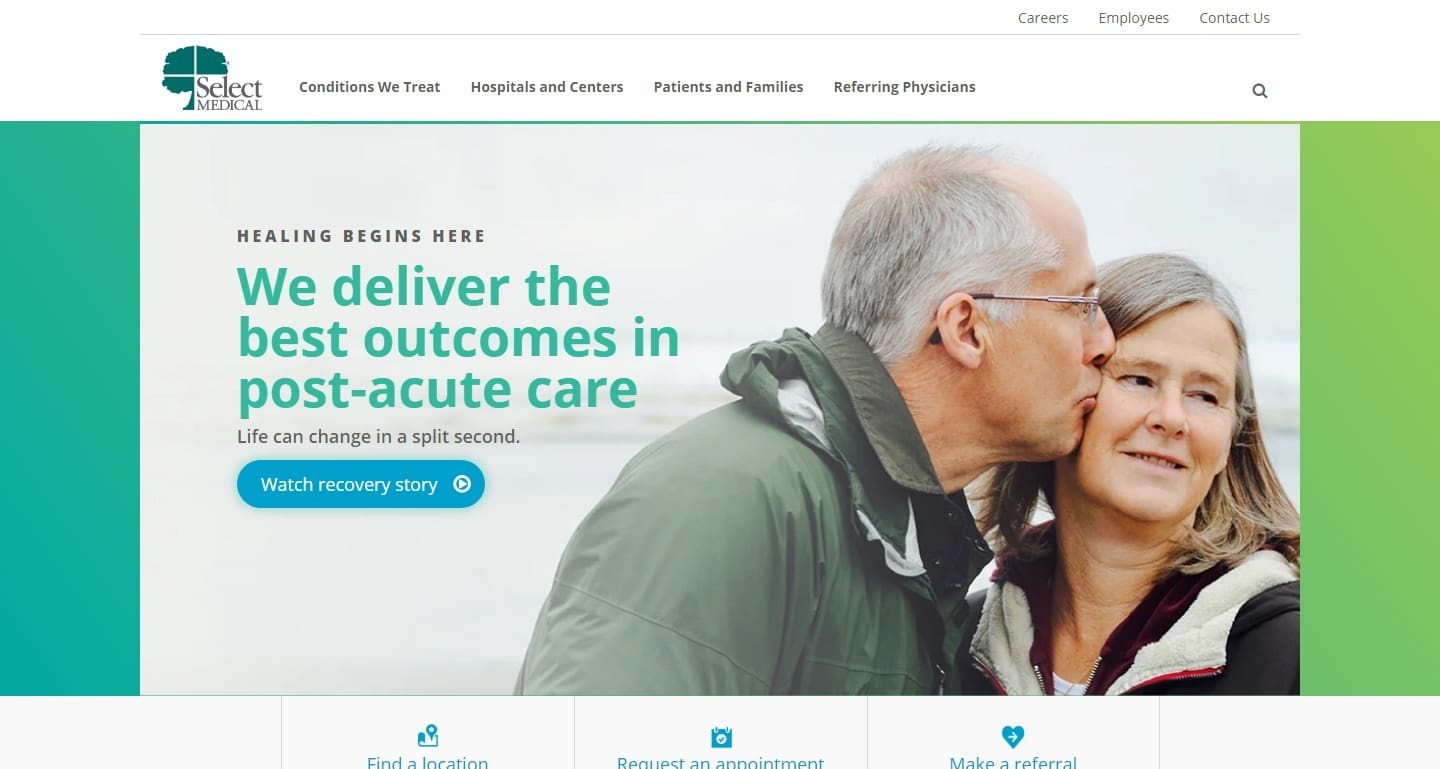This screen recording captures the homepage of a website dedicated to medical services. At the top of the page, there is a navigation bar featuring sections titled "Careers," "Employees," and "Contact Us" in gray text, separated by a thin gray line. Below this, the website's logo—a green tree—is prominently displayed alongside the name "Select Medical" in gray text.

The main navigation menu outlines key sections: "Conditions We Treat," "Hospitals and Centers," "Patients and Families," and "Referring Physicians," alongside a gray magnifying glass icon for search functionality. Immediately below this menu, a large, eye-catching image occupies much of the screen, set against a green and teal backdrop with a predominantly white background. The image depicts an older couple; the woman, dressed in a black jacket with gray hair, is being kissed on the cheek by her husband, who has glasses, gray hair, and an olive jacket.

Overlaying the image is a motivational message in a combination of teal and black fonts: "Healing begins here. We deliver the best outcomes in post-acute care. Life can change in a split second." Below this message, a blue box with white text invites users to "Watch Recovery Story," featuring a play button icon.

Towards the bottom of the page, there is a section with teal-colored icons on a gray background. The first icon, resembling a location pin, includes the text "Find a Location." The second icon, resembling a calendar with a check mark, reads "Request an Appointment." The third icon, a heart with a white arrow, is labeled "Make a Referral." The visual quality of the page is exceptionally clear, with large, user-friendly fonts that are accessible and easily readable for users with low vision.